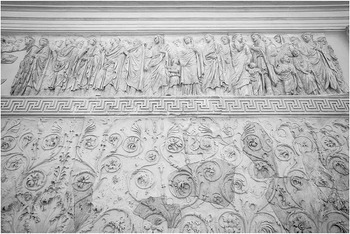This close-up photograph captures the intricate details of a portion of the Colosseum in Rome, showcasing its elaborate ornamentation. The wall, predominantly white with hints of gray, features ornate carvings and etchings. At the base, there are scrolling patterns resembling 'S' shapes and floral designs, including roses, which are raised off the plaster surface. Above this section is a horizontal bar adorned with a complex geometric pattern. The topmost layer displays a frieze of men, likely from the Greek period, carved in a variety of toga-like robes and some wearing wreaths. The figures are arranged shoulder-to-shoulder, with differing postures and directions, some standing, others kneeling, and all intricately detailed despite the small scale. This detailed craftsmanship highlights the rich decorative elements typical of ancient Roman architecture.